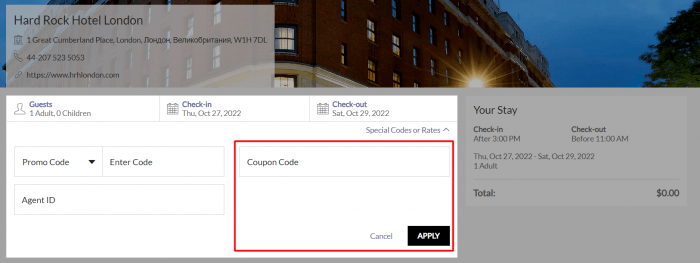Screenshot from a booking site for the Hard Rock Hotel in London. Displayed at the top is the address:

One Great Cumberland Place, London, W1H 7DL, with the rest of the address in Russian. The contact number provided is +44 207-523-5053, and the website listed is HRHLondon.com.

Below these details, there is a white field for booking specifics that indicates:
 
- Guests: 1 adult, 0 children
- Check-in: Thursday, October 27, 2022, after 3 p.m.
- Check-out: Saturday, October 29, 2022, before 11 a.m.
- Total cost: $0, suggesting this is a test screen
- Options for promo code, intercode, and agent ID are present but not selected, while the coupon code field is highlighted with a red outline. The cancel and apply buttons are situated below this field.

Outside this booking section, the background shows an external view of the Hard Rock Hotel from the sidewalk. The image captures the brick facade of the building at a corner, displaying both its front and side.